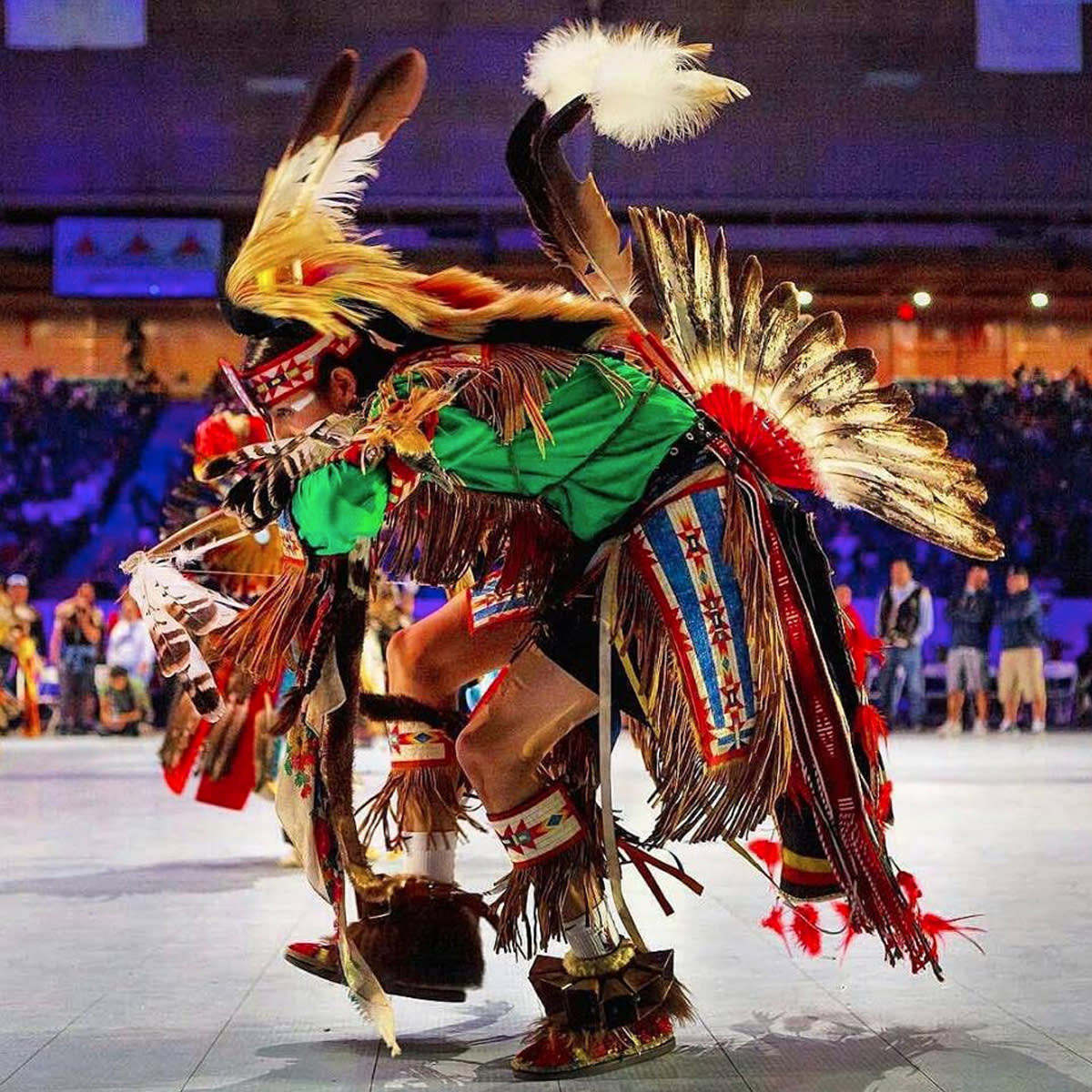The image captures a dynamic stage performance indoors, possibly within a concert hall, auditorium, or school venue, characterized by its dark backdrop illuminated with purple hues. The focal point is a central performer adorned in vibrant Native American regalia, richly embellished with feathers of yellow, red, and brown, and intricate woven banners in blue, white, and red. The performer wears a green shirt, black shorts, golden leggings, and brown boots, complemented by a dramatic headgear featuring horns, feathers, and ornamental elements resembling tails and wings. Surrounding the main performer, other blurred figures stand ready in the background, amidst the audience's presence visible in the dimly lit stands, contributing to the festive atmosphere of the event.